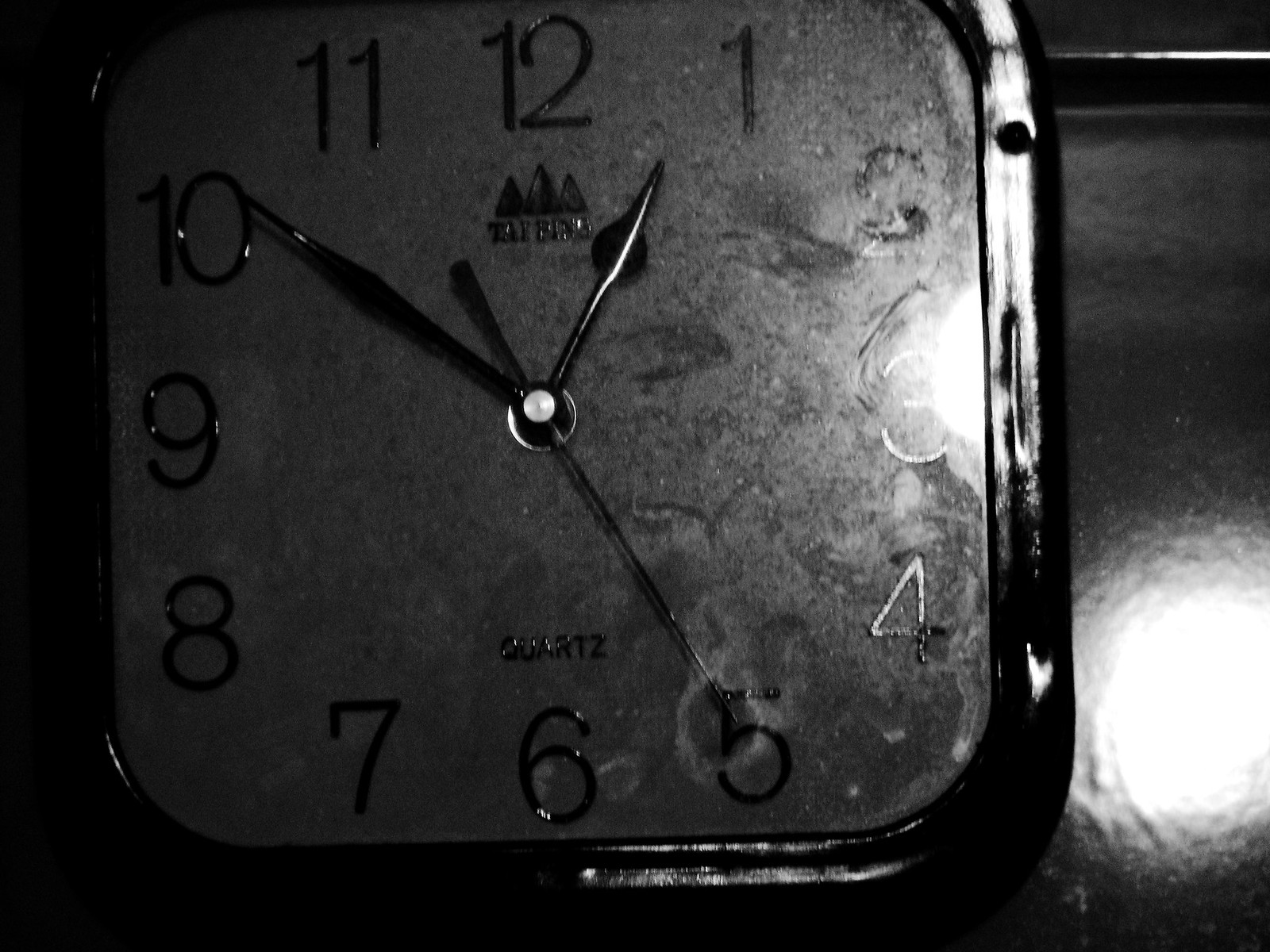A detailed black and white image of a watch face in low light conditions. On the very right edge of the timepiece's face, there's a reflection of a bright white light, which is also mirrored at the edge of the image. The backdrop is a dark color, providing a stark contrast to the timepiece. The watch face itself appears to be a dark gray color, featuring black letters and numbers. The clock's hour, minute, and second hands are dark, likely black, and are centered with a silver fastener. An icon depicting three evergreen trees is situated just under the 12 o’clock mark, along with an obscured brand name, blending into the reflected light. Near the bottom of the face, just above the 6 o’clock position, the word "QUARTZ" is inscribed in black.